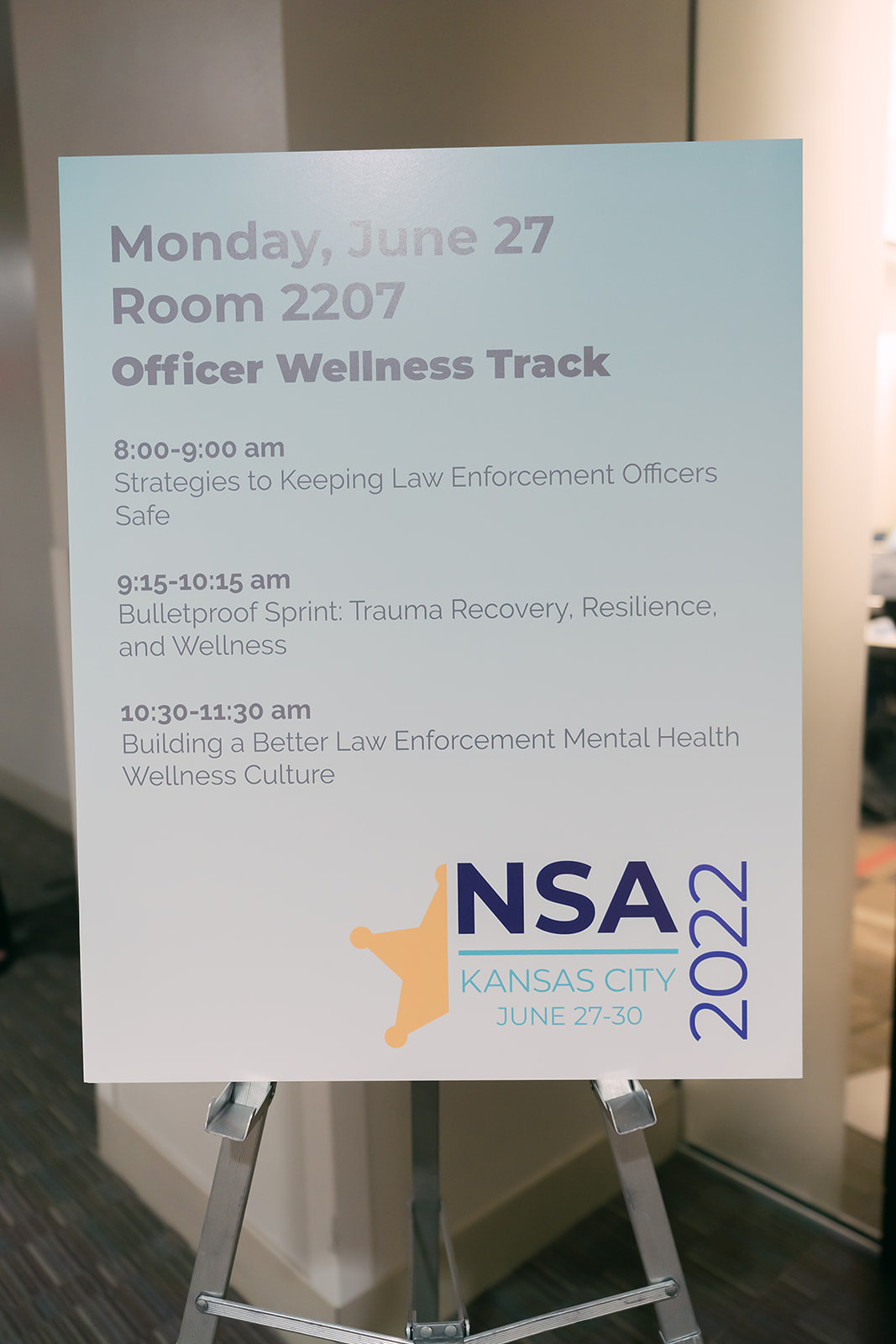In this image, we see a detailed poster mounted on a steel-colored metal easel, displayed indoors on commercial carpeting typical of hotel hallways. The sign, designed with a faded sky blue top transitioning to white at the bottom, lists a series of sessions for an Officer Wellness Track conference. The header, written in bold light gray, announces the date as "Monday, June 27th," and the location as "Room 2207." Below the header are the session details: "8 to 9 a.m. - Strategies to Keep Law Enforcement Officers Safe," "9:15 to 10:15 a.m. - Bulletproof Sprint, Trauma Recovery, Resilience, and Wellness," and "10:30 to 11:30 a.m. - Building a Better Law Enforcement Mental Health Wellness Culture." At the bottom right corner of the poster, the conference logo features "NSA" in large dark blue letters, accompanied by a half-star sheriff's badge icon, and the words "Kansas City, June 27-30, 2022." The poster catches some glare from the overhead lighting, highlighting its professional setting near a white-walled room and door.